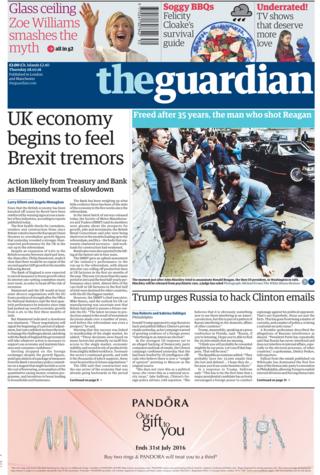The image depicts the front cover of a Guardian newspaper. In the top left corner, there is a headline featuring Hillary Clinton with the text, "Glass ceiling: Zoe Williams smashes the myth." Adjacent to this on the right, a headline reads "Soggy barbecues: Felicity Cloak's survival guide." Further to the right, another headline highlights "Underrated TV shows that deserve more love."

Below these sections, there is a dark blue box that prominently displays "The Guardian." Beneath this title, a headline reads, "UK economy began to feel Brexit tremors; action likely from Treasury and Bank, Hammond warned of slowdown."

A significant portion of the front page is dominated by a photograph showing several people lying on the sidewalk, surrounded by a few cars and a group of onlookers. The caption under the picture states, "Freed after 35 years: the man who shot Reagan."

Another headline below the photograph reads, “Trump urges Russia to hack Clinton emails.”

At the bottom of the cover, there is a pink box with the text, "Pandora: our gift to you."